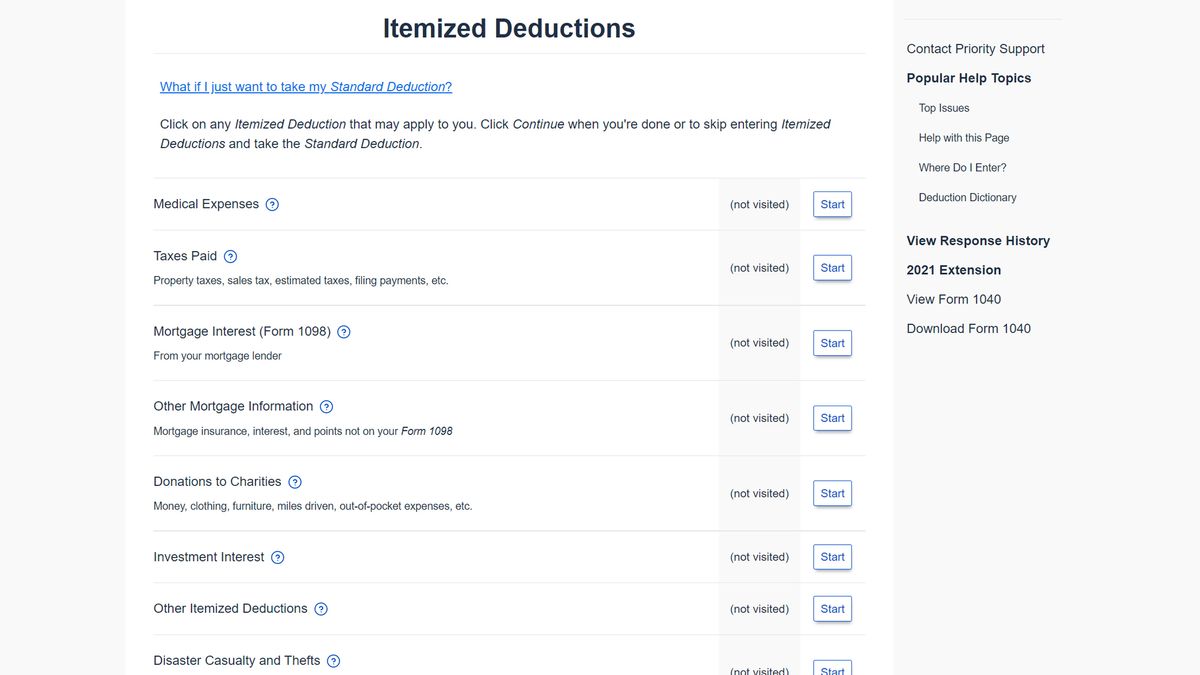The webpage layout features a comprehensive interface designed to assist users with their tax-related queries and tasks. 

### Right-Hand Side 
The right-hand side of the page is framed by a dark grey bezel. At the top, there is a dropdown menu labeled "Contact Priority Support." Below that is a section titled "Popular Help Topics" in bold black text. This section is subdivided into several topics:

1. Top Issues
2. Help with the Page
3. Where Do I Enter
4. Deduction Dictionary 

Further down, another section titled "View Response History" is displayed in bold black text, followed by "2021 Extension." Below this, there are non-bold options for "View Form 1040" and "Download Form 1040."

### Left-Hand Side
On the left-hand side, bold black text reads "Itemized Deductions." Under this, in a lighter grey area, there is a hyperlink in blue that says, "What if I just want to take my standard deduction?" 

Further down, another bold black text instructs: "Click on the itemized deductions that may apply to you. Click Continue when you have done or to skip the entered itemized deductions and take the standard deduction."

Each itemized deduction category is listed below, starting with "Medical Expenses" and accompanied by a blue question mark icon. To the right of each category is a large rectangular area in dark grey indicating the status, currently stating "Not Visited." Next to each status box is a small white button with a blue border and text that says "Start."

The categories listed are:
1. Medical Expenses
2. Taxes Paid: Property taxes, sales tax, estimated tax, filing payments, etc.
3. Mortgage Interest (Form 1098 from your mortgage lender)
4. Other Mortgage Information
5. Mortgage Insurance, Interest, and Points Not on Form 1098
6. Deductions to Charities: Money, clothing, furniture, miles driven, out-of-pocket expenses, etc.
7. Investment Interest
8. Other Itemized Deductions
9. Disaster, Casualty, and Thefts

Each category is intended to guide the user through the process of entering information relevant to itemized deductions with clear indicators and action buttons.